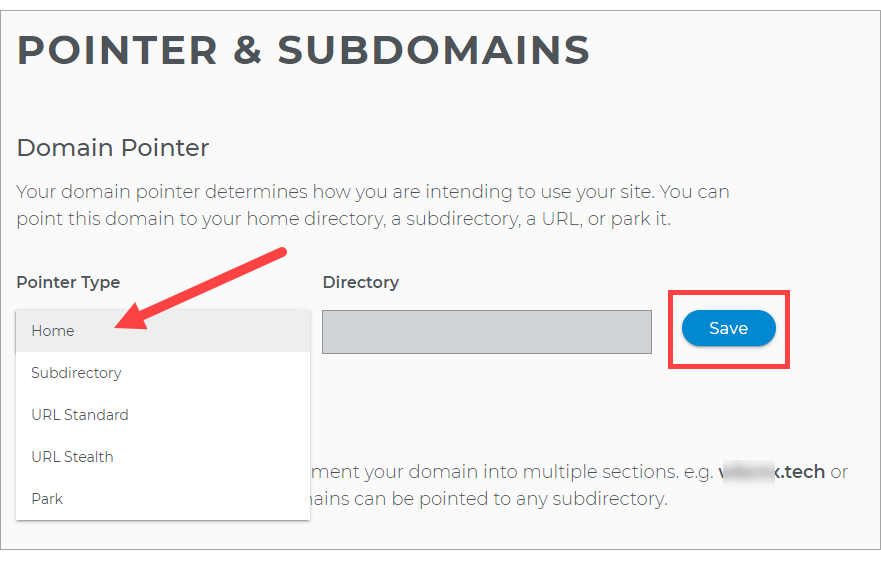The image is horizontally rectangular with a very light grey background framed by a thin dark grey to black border. At the top left, in large, bold, all-capital letters, it reads "POINTER AND SUBDOMAINS." Below this title, in smaller, normal font, it says "Domain Pointer," followed by a description in light grey lettering: "Your domain pointer determines how you are intending to use your site. You can point this domain to your home directory, a subdirectory, a URL, or park it."

On the left side of the image, there is a label "Pointer Type" accompanied by a drop-down menu. The drop-down menu features an overlay of a large arrow pointing to the first selection, "Home." The other options listed are "Subdirectory," "URL Standard," "URL Stealth," and "Park."

To the right of this dropdown, there is another label "Directory" next to an input field where users can specify the directory. Further to the right, there is a prominent blue "Save" button outlined by a red horizontal rectangle border. The overall design of the interface is clean and functional, guiding the user through the process of setting up their domain pointer.